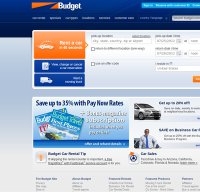In the image, a webpage is displayed, but the text appears slightly blurred. At the top, the header has a dark blue background with a logo combining orange and blue hues on the left. Adjacent to the logo is the word "Budget" in white font. Centrally placed in the header is a prominent message in blue text that reads: "Save up to 35% with Pay Now Rate." Although some surrounding words are not legible, checkboxes accompanied by colors interspersed with orange and blue details can be seen.

On the right side of the page, there's an image of a silver-gray car. Below this, another image features a person casually leaning against a car, dressed in a white t-shirt and a blue tie. At the bottom of the page, there's a text banner with the words "Budget Car Rental Tip" in blue, but the specific text on the bottom left corner is partially obscured and difficult to discern.